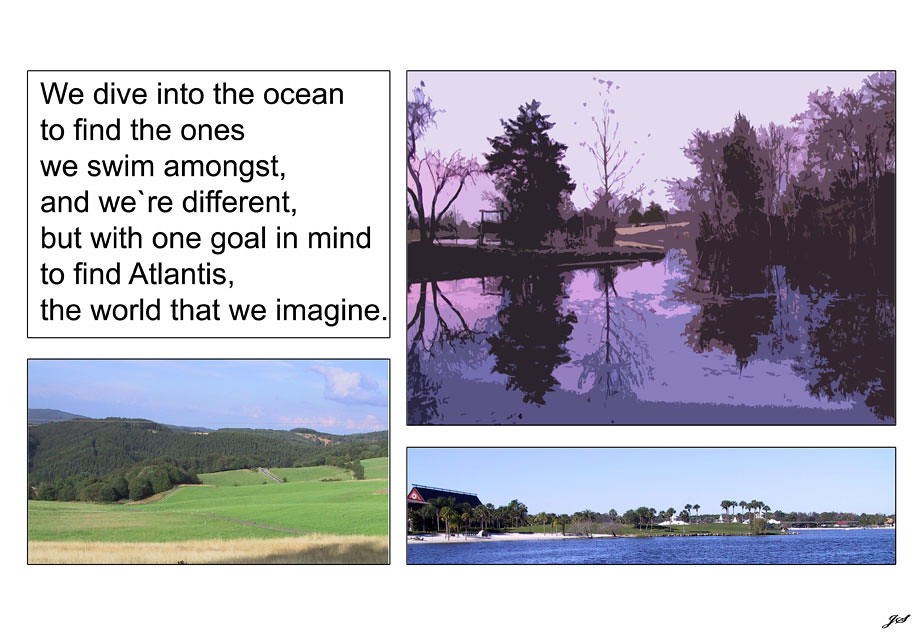The composite image is a mixed-media graphic with elements resembling a comic strip, featuring a combination of real photographs and digitally created elements. The layout is divided into four sections, each separated by black borders.

On the top left, there is a text box containing the motivational phrase: "We dive into the ocean to find the ones we swim amongst, and we are different, but with one goal in mind – to find Atlantis, the world that we imagine."

Directly below the text, occupying the bottom left corner, is a serene landscape photograph. This image captures a bright, sunny day with a clear blue sky scattered with white clouds. The foreground features a verdant green field with tall trees that ascend a hillside or small mountain. The area is lush with greenery and includes pathways and possibly bridges, suggesting it's a farm or park area. Shadows cast by the sunlight indicate the daytime setting.

On the top right side of the composite, there is a digitally painted scene depicting a tranquil body of water that resembles a lake. This water is a deep blue and reflects its surrounding trees, which appear dark and somewhat blackened, set against a sky with gray or purple hues.

Below this painting, in the bottom right section, lies another photograph showcasing a cleaner water body, possibly a river or another lake. This water is a vibrant blue, bordered by a mix of green grass and palm trees. A building that looks like a hotel or resort sits near the shore, with other scattered structures visible in the background. The scene is under a clear blue sky, indicating a bright and sunny daytime setting. The bottom right of this photo is signed "GED," presumably the artist or photographer's initials.